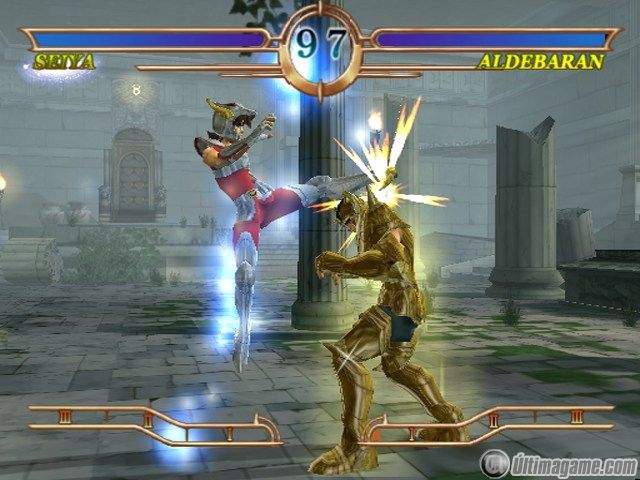The screenshot depicts an intense moment from a fighting video game. The names "Seiya" and "Aldebaran" are displayed at the top left and top right corners, respectively. A timer at the center top shows "97." The health bars, featuring a purple-blue gradient, are prominently positioned near the top.

The central character is a woman outfitted in a unique mix of futuristic and primitive attire. She wears red spandex and dons a headpiece resembling an animal skull, complete with two prominent tusks or horns. Her legs and waist are wrapped in metallic bands, enhancing her battle-ready appearance. Caught mid-action, she is airborne with one leg extended in a powerful kick aimed at a man clad in gleaming golden armor, who appears to be recoiling from the impact. Sparks erupt from the point of contact, accentuating the fierce exchange.

Golden bars are scattered throughout the frame, possibly signifying special items or power-ups. At the bottom of the screen, a series of Roman numerals (I, II, III) likely indicate levels or stages of the fighting meter. The bottom right corner features the website "UltimaGame.com" alongside the Ultima logo, suggesting this is a promotional or in-game display.